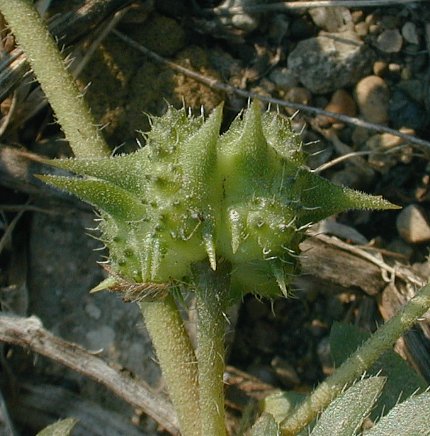The image showcases a lime green, spiky succulent, likely a type of cactus, situated prominently in a rocky outdoor setting. The plant, not a typical cactus in appearance, features a blobby main bud with several spikes of varying sizes—larger spikes dominate while numerous smaller ones fill in the gaps. It is composed of three stems: two attached directly to the main bud and one positioned at the bottom right corner. All stems are covered in tiny hairs. The succulent is centered in the photograph, which also captures a variety of background elements, including dirt, gravel, branches, and a significant rock on the left side of the image. The plant's color is a muted green, adding to the natural ambiance of the scene.